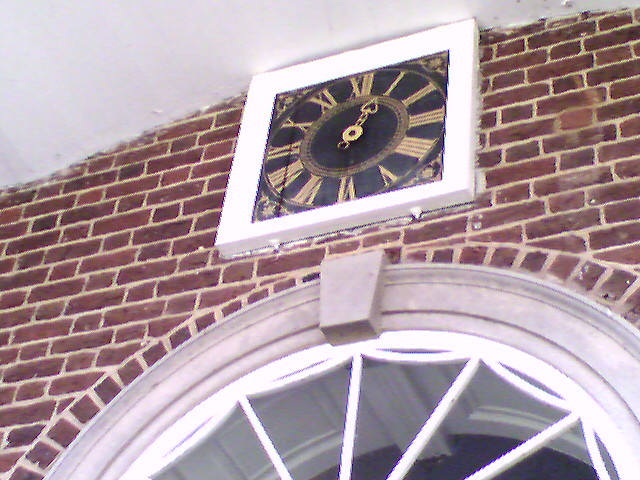The image features a room with a richly textured and architecturally complex scene. At the top of the image, a white-painted ceiling forms a clean, spacious backdrop. Dominating the middle portion is a striking brick wall, showcasing a gradient of red hues interspersed with white and cream mortar lines adding depth and character. Mounted at the top of this brick wall is an elegant clock encased in a white frame. The clock itself is a sophisticated piece, designed in black and gold, with Roman numerals marking the hours. A gold arrow hand points precisely to the one o'clock position. Towards the bottom, the bricks form a semi-circular pattern, leading the eye to a cream-colored element that appears to be part of a white architectural structure, perhaps a table or cabinet. This structure features intricate black and white components, creating an intriguing contrast and adding further detail to the scene.